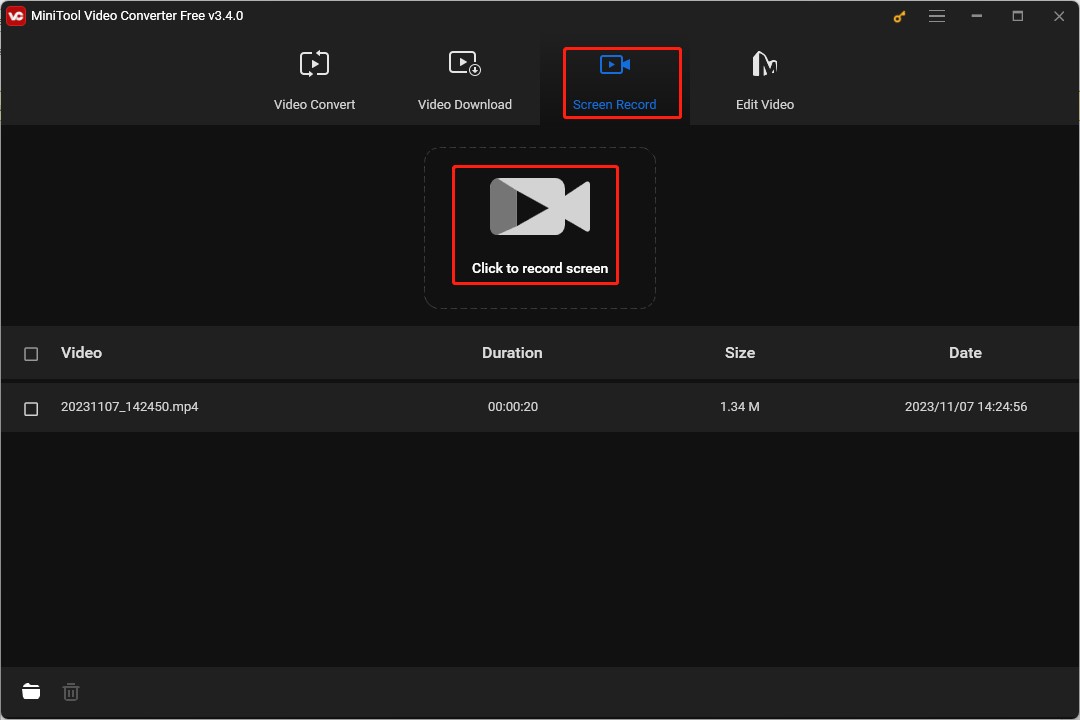This is a detailed screenshot of the user interface of MiniTool Video Converter Free, version 3.4.0. The top section of the interface features a dark gray navigation bar with the following options arranged from left to right: "Video Convert," "Video Download," "Screen Record" (which is currently selected and highlighted with a red box), and "Edit Video." 

Centrally located beneath the navigation bar is a prominent red box displaying an icon of a video camera with the text "Click to Record Screen," indicating the functionality to initiate a screen recording.

Further down the interface, there are two horizontal gray bars, each spanning the width of the screen. On the left side of each bar is a small empty square checkbox. The first bar is labeled "Video," and underneath, it specifies the file format as MP4. Adjacent to this, the description field consists of multiple zeros followed by ".00." The size of the file is noted as "1.34 MB," and finally, the date and time stamp "2023-1107-1424.56" is provided.